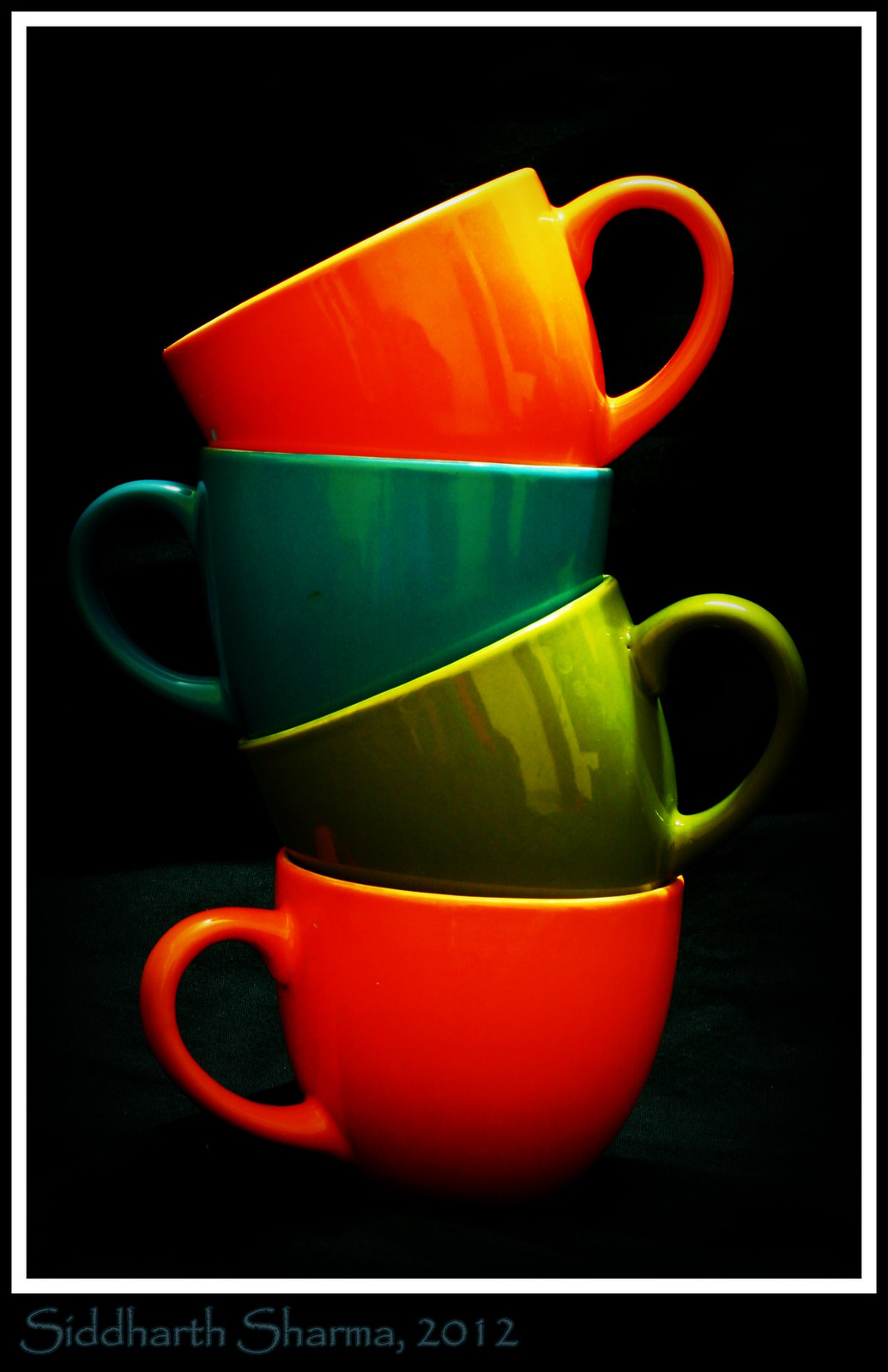This photograph, likely taken by Siddharth Sharma in 2012, captures a striking arrangement of four coffee mugs against a black background with subtle green lighting near the base. The mugs are stacked in alternating positions, with the handles oriented in opposite directions: the bottom cup, dark orange or red, has its handle to the left; the second cup, green, has its handle to the right; the third cup, blue, has its handle to the left; and the top cup, matching the bottom in color, has its handle to the right. Notably, the image's composition highlights alternating tipping orientations of the cups, enhancing the visual intrigue. The photograph is framed in white, and light reflections add a touch of realism, particularly on the top orange and middle green mugs. At the bottom of the image, the photographer's name, "Siddharth Sharma 2012," is elegantly inscribed in blue text.